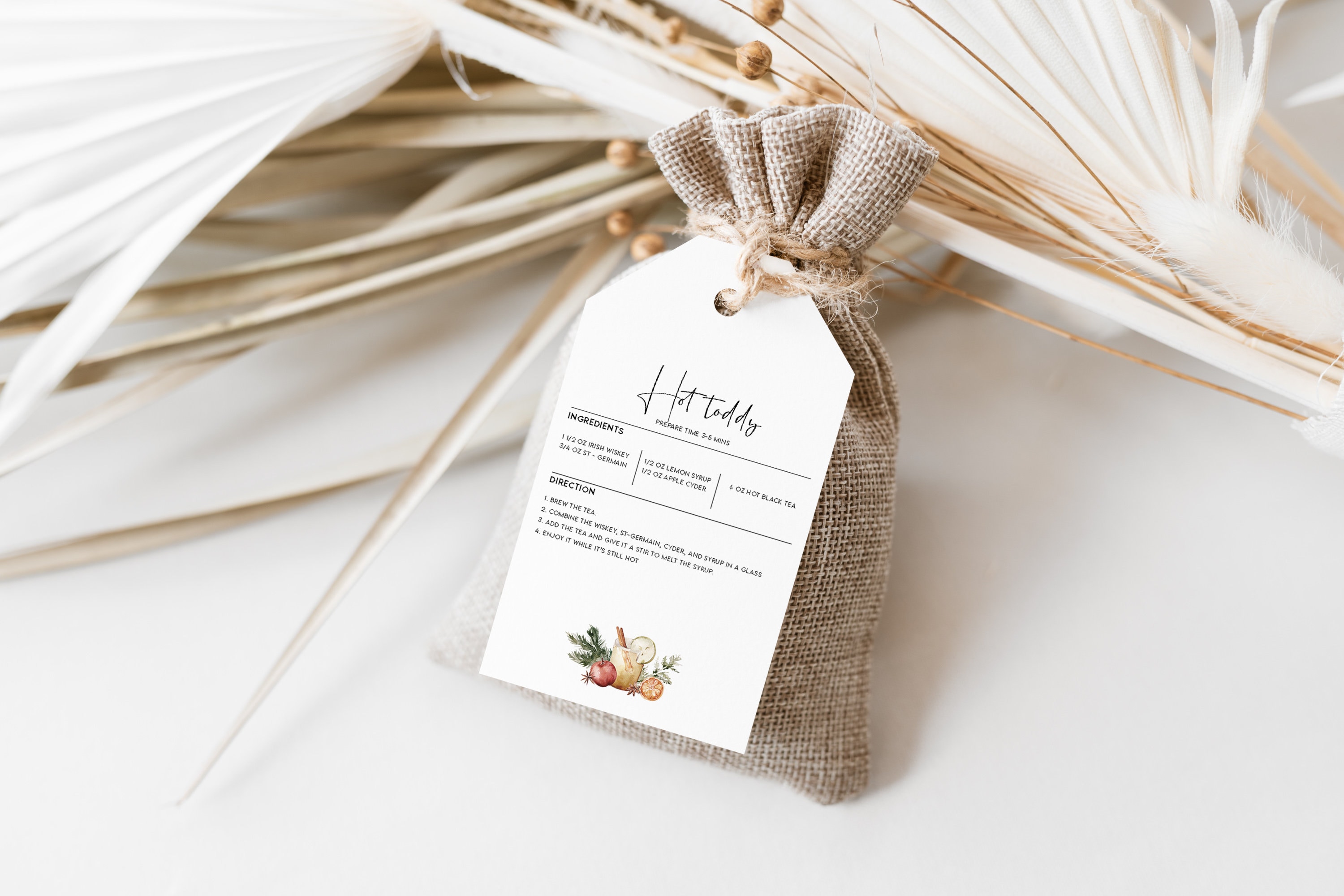This photograph resembles a curated Instagram image. At the center, a small burlap sack tied with twine is featured prominently, almost entirely covered by a large, white tag. The tag, inscribed in detailed script, prominently reads "Hot Toddy," followed by preparation instructions and an ingredient list. The ingredients include one and a half ounces of Irish whiskey, three-fourths ounces of St. Germain, half an ounce of lemon syrup, half an ounce of apple cider, and six ounces of hot black tea. The preparation steps are: brew the tea, combine the whiskey, St. Germain, cider, and syrup in a glass, add the tea, stir to melt the syrup, and enjoy while hot. The background consists of soft, white feathery foliage and tan, wheat-like dried flowers arranged behind the sack, all positioned on a white table, enhancing the natural and rustic aesthetic of the setup.